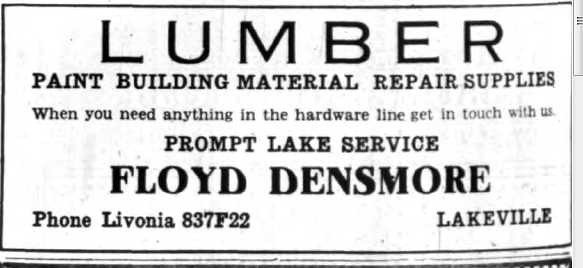This black-and-white image appears to be an old advertisement, perhaps a clipping from a newspaper or a small label, with dimensions approximately 3 inches tall by 6 or 7 inches wide. At the top, in large capital letters, it boldly reads "LUMBER." Below this, in slightly smaller capital letters, the text lists "PAINT BUILDING MATERIAL REPAIR SUPPLIES." Centered beneath these lines is a sentence in small lettering that states, "When you need anything in the hardware line, get in touch with us." Following this, in capital letters matching the size of the previous line, it reads "PROMPT LAKE SERVICE." Further down, in large bold letters, the name "FLOYD DENSMORE" is prominently displayed. In the bottom left corner, the contact information is presented as "PHONE LAVONIA 837-F22," while in the bottom right corner, the location "LAKEVILLE" is indicated. This layout and the style suggest it is an advertisement from a bygone era, representing Mr. Densmore's hardware business in Lakeville.